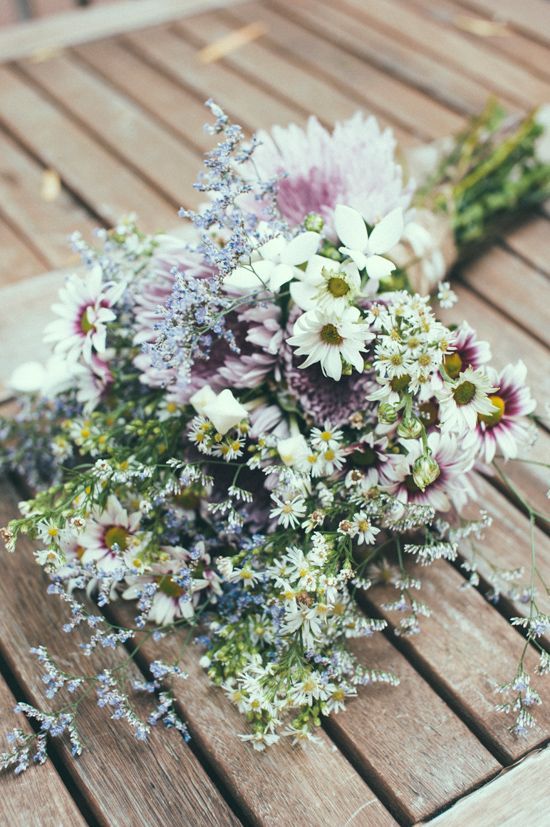The image captures a rustic-looking bouquet of flowers lying on its side atop light brown wooden slats, which could be a deck, boardwalk, or bench. The bouquet includes a variety of flowers: small white ones with green or yellow centers, white flowers with purple interiors, and some purple mum-like and tiny light blue flowers, all bundled together in a makeshift, country-inspired arrangement. The photograph appears professional, featuring a shallow depth of field that softens the background and emphasizes the bouquet's details, including the visible green stems and the brown wrap tying them together. The bouquet, with its blend of whites, purples, greens, and yellow centers, exudes a charming yet understated beauty.